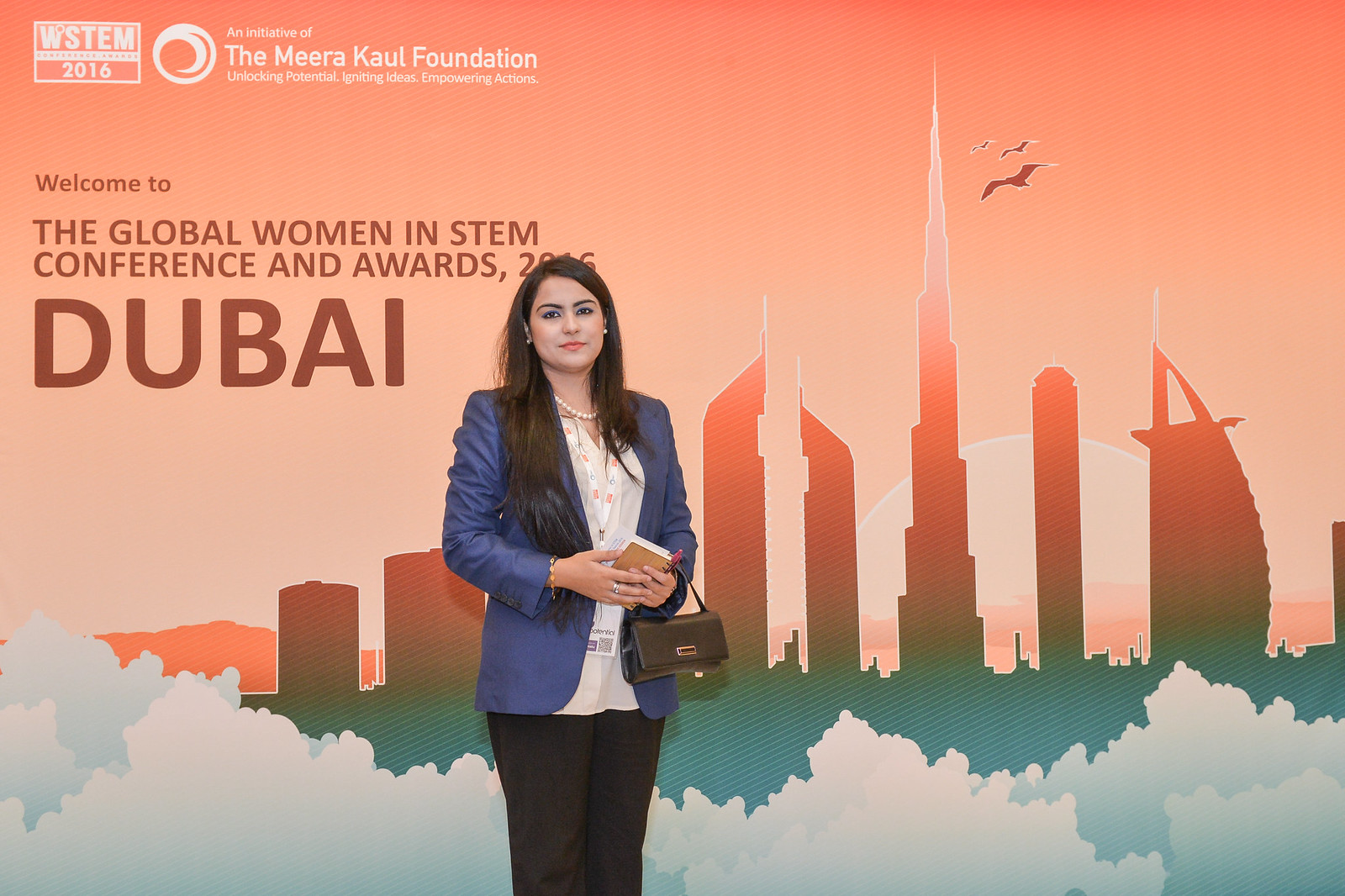The image depicts a woman standing slightly left against a large, cartoonish backdrop showcasing a city skyline with various skyscrapers transitioning from pink at the top to blue at the bottom, and white clouds below. The sky features shades of orange and turquoise, with small birds flying and a hint of a sunrise or sunset. The sign behind her reads "WSTEM 2016, an initiative of the Miracal Foundation, unlocking potential, igniting ideas, empowering actions. Welcome to the Global Women in STEM Conference and Awards 2016 in Dubai" in white and red font.

The woman has long dark hair cascading to her waist, light skin, and is adorned with red lipstick, earrings, a pearl necklace, and a lanyard with a badge around her waist. She is dressed in a light-colored blouse under a blue blazer, and black pants. She holds a notebook in one hand and her left wrist carries a black purse. Her attire is complemented by a bracelet and rings, creating a polished and professional look. 

The backdrop's vibrant hues of black, peach, red, various shades of pink, gray, green, blue, white, gold, and multiple shades of white and gray contrast vividly with her ensemble, making her the focal point of the image.